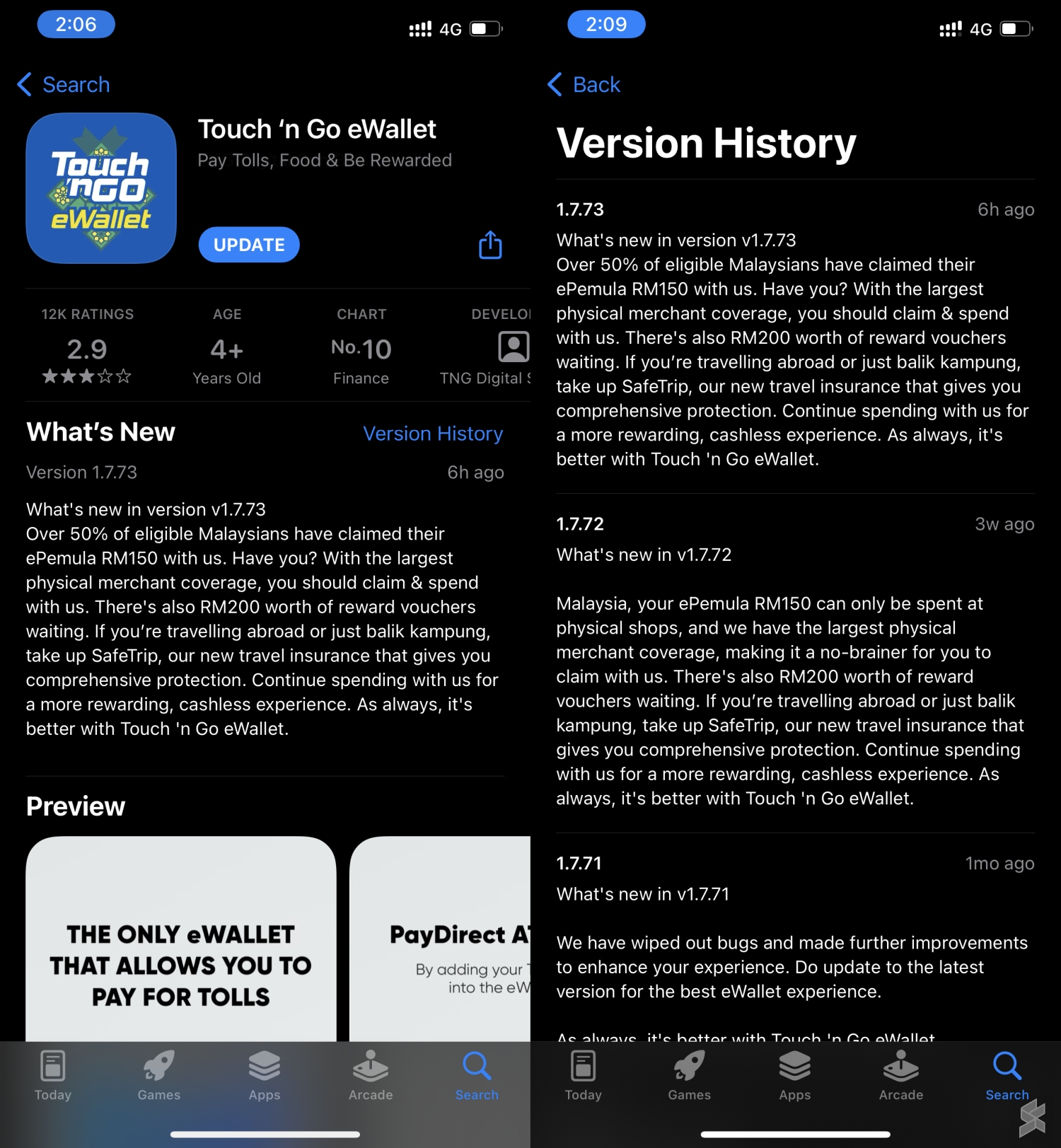A smartphone screen displaying an app version update notification for the Touch 'n Go E-Wallet. In the status bar, the time reads 2:06 PM, accompanied by various status icons including data connection, 4G, and a half-full battery indicator. Below, a prominent blue clickable 'Search' button is visible. The update notification details various features such as "Touch 'n Go E-Wallet: Pay tolls, buy food, and earn rewards" with an update button underneath.

Further below, the app details show 12K ratings at 2.9 stars, an age rating of 4+, and its ranking as #10 in the finance category. It is developed by TNG Digital. The "What's New" section for version 1.7.7.3 highlights that over 50% of eligible Malaysians have claimed their RM150 E-Pemil incentive with the app, urging users to claim and spend with the largest physical merchant coverage available. Additionally, RM200 worth of rewards vouchers are offered. The new travel insurance feature ensures comprehensive protection whether traveling abroad or locally ("balik kampung").

The update encourages continuing use of the app for a more rewarding, cashless experience, and emphasizes that Touch 'n Go E-Wallet is the only e-wallet enabling toll payments. A reiterated reminder on the far right-hand side highlights previous updates about bug fixes and improvements, urging users to download the latest version for the best e-wallet experience.